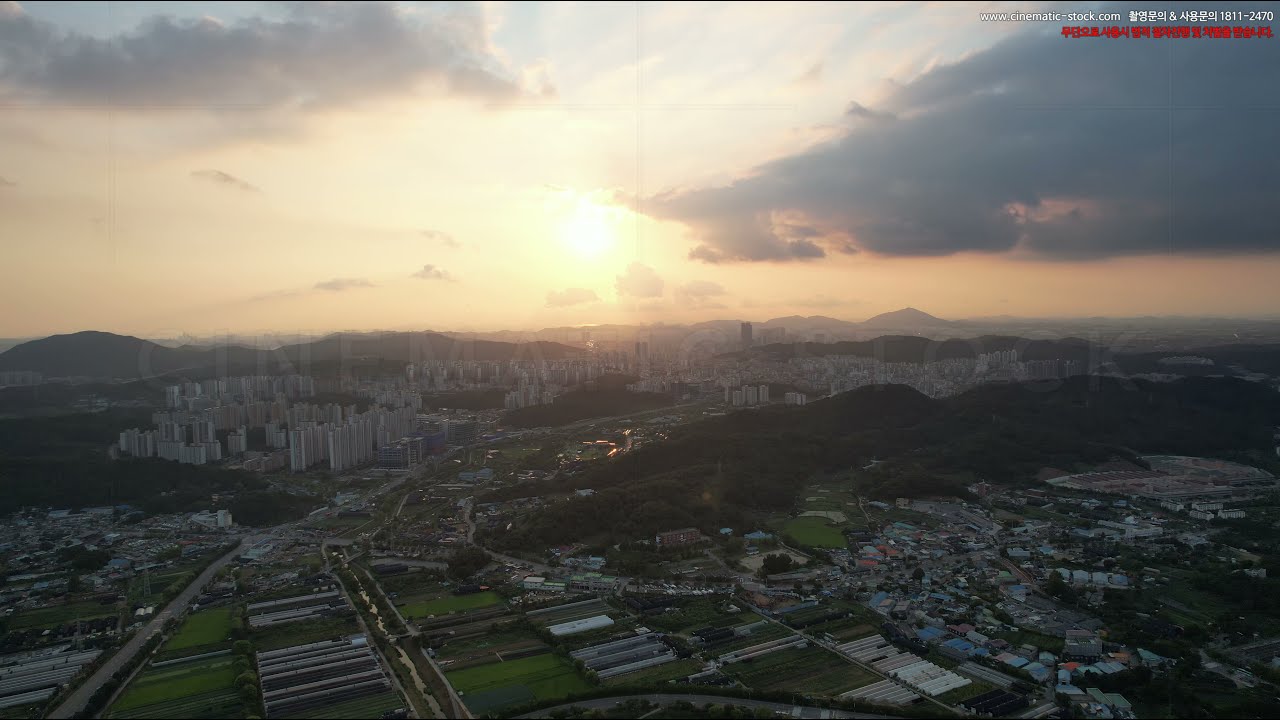This aerial photograph captures a sprawling city at sunset, taken from a high elevation, possibly by a drone or plane. The rectangular image showcases various city elements under a cloudy sky tinged with shades of orange, yellow, and brown from the setting sun. In the background, hills and mountains can be seen, acting as a natural barrier between different parts of the city. 

On the right side of the image, residential areas with clusters of houses and apartment buildings are visible. Moving leftward, an industrial or agricultural zone with green patches and several buildings stands out, possibly indicating greenhouses or farm operations. A main road transverses this area, leading off into the background.

The center of the image is dominated by a collection of skyscrapers and condos, suggesting a busy metropolitan zone. Despite the cloud cover, the bright reflection of the sun remains noticeable, hidden behind the big gray cloud in the top right corner. 

Overall, the photograph offers a detailed and comprehensive view of the city’s diverse landscape, illuminated by the warm hues of the setting sun, with text in the upper right corner indicating it's stock footage from www.cinematic-stock.com, accompanied by Japanese or Chinese characters.